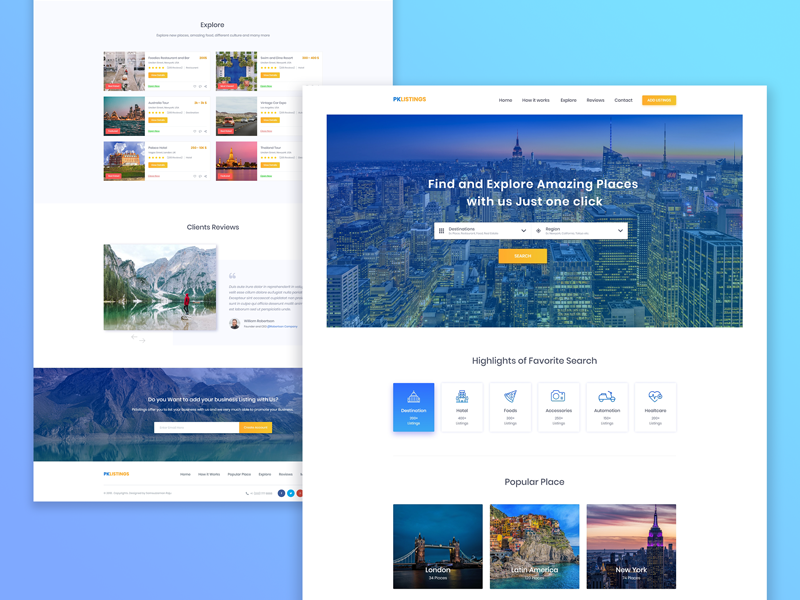The image features a screen divided into several distinct sections. The top portion of the screen features a turquoise background that stretches from slightly left of center all the way across the top and down the right-hand side. On the left side, there is a narrow vertical column in periwinkle blue, approximately an eighth of an inch wide. This blue strip extends downwards before continuing horizontally, covering nearly half the screen in the same periwinkle shade.

Central to the screen's design are two vertical white rectangles. The smaller rectangle on the left is partially overlapped by the larger one on the right. The smaller rectangle spans roughly a quarter of the screen from about a third of the way down to the bottom. It contains six small images arranged in two columns and is labeled "Clients to Review," although the text is barely legible.

The larger white rectangle on the right is more detailed. At the top, it features an animated image of a city within a horizontal vertical box. Overlaid on this image is white text that reads, "Find and explore amazing places with us, just one click." Below this animation, there's a horizontal white box featuring additional text that says, "Highlights of Favorite Search." This section includes several vertical boxes, each marked by a blue icon and accompanying text, though the text is too small to discern.

Toward the lower part of this larger rectangle, there’s a section labeled "Popular Places" displaying three vertical images in separate boxes. The first box is labeled "London," the second "Latin America," and the third "New York," each showcasing scenes representative of these locations.